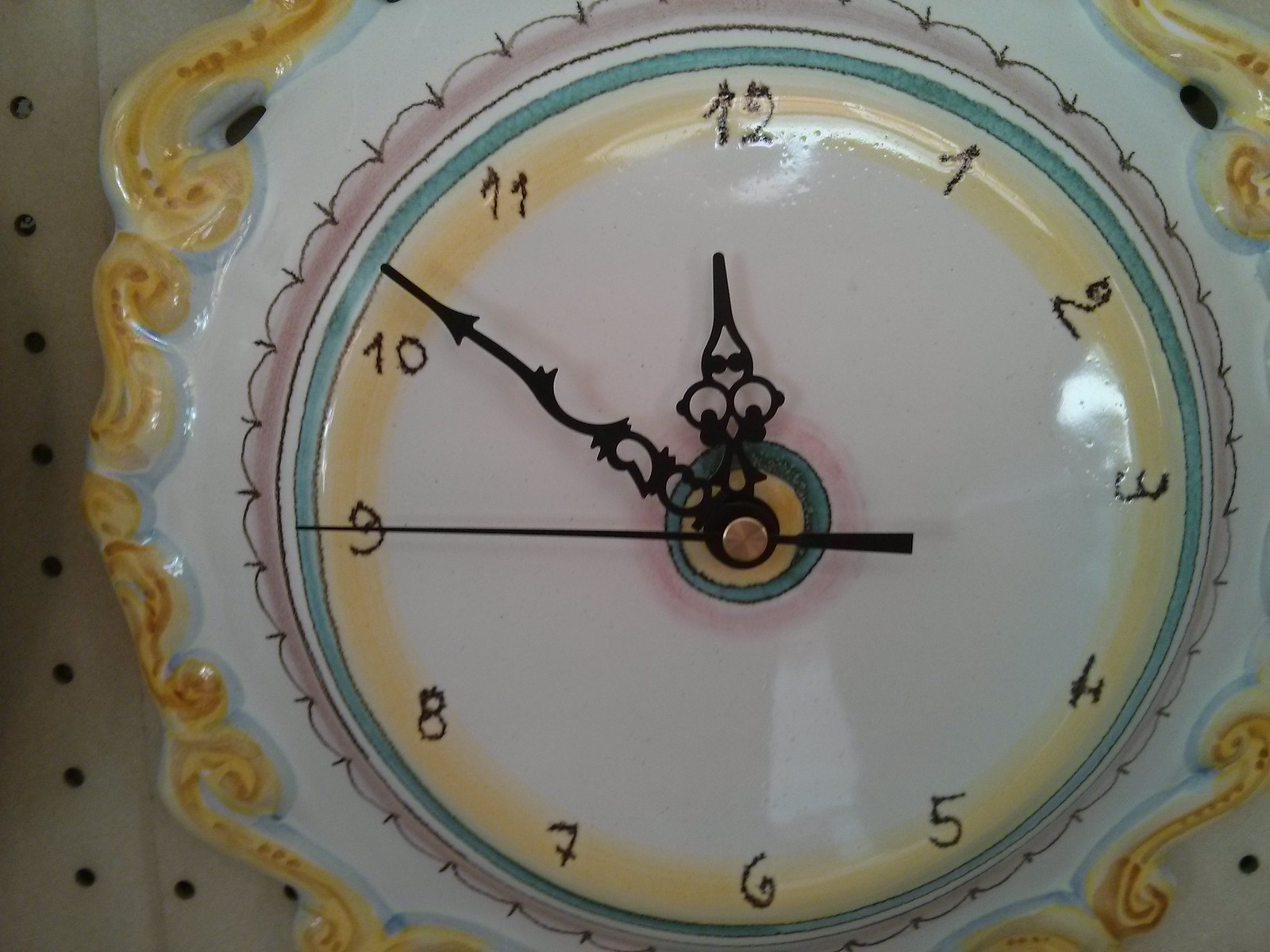This rectangular, horizontally-oriented image showcases an exquisite, handcrafted pottery clock. The clock's base is a pristine white, adorned with an ornate yellow scroll design that frames the timepiece. At the heart of the clock is a circular blue face, with black, hand-painted numbers artfully arranged. The clock's time reads 11:52, indicated by two large black hands featuring an elegant scroll design. A narrow black second hand points towards the nine. Adding a touch of subtle sophistication, intricate pink scrollwork nestles between the blue central circle and the encompassing yellow scroll, highlighting the intricate craftsmanship of the piece.